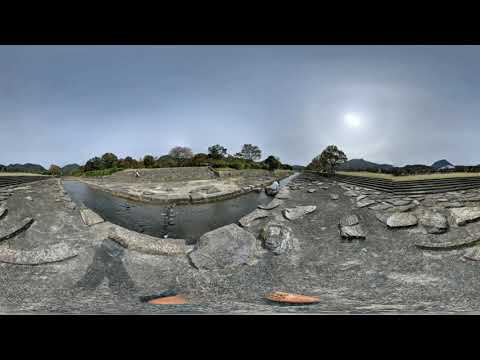This panoramic, 360-degree outdoor image reveals a natural environment rich with geological and arboreal details. Dominated by rugged, grayish rocks, the scene presents a striking river or canal running horizontally through the center, with the waterway giving the illusion of curving due to the panoramic nature of the shot. The banks of the water feature stone formations on either side, some of which exhibit a subtle pink hue, contrasting with the more common light gray tones.

On the upper right side of the image, a dense line of tall, dark green trees creates a lush backdrop, standing further back from the rocky shore. Toward the right edge, one can also discern the presence of a staircase, suggesting human interaction with the landscape. The sky above is a light, early autumn blue, sporadically dotted with clouds, adding a serene atmosphere to the scene.

Despite a somewhat distorted perspective, the image captures a clear, bright daylight setting, vividly highlighting the natural and potentially man-made elements of the area. The overall color palette includes various shades of blue, gray, green, with touches of orange and pink, effectively emphasizing the diverse textures and formations within this picturesque outdoor scene.